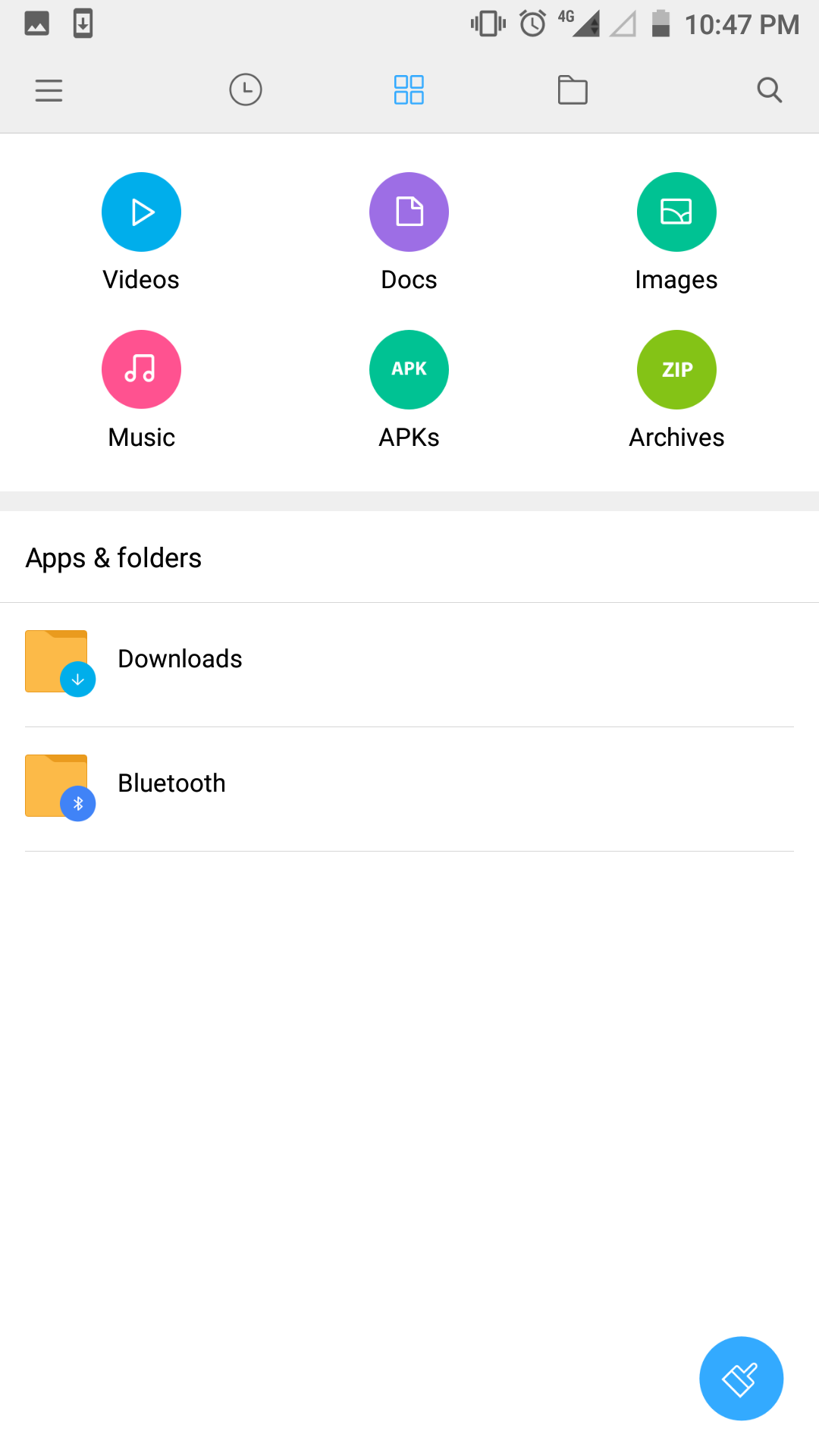This image captures the screen of a smartphone displaying various application icons. At the very top, a gray notification and status bar contains several icons: on the left is a cell phone symbol, while on the right, there's a clock showing the time as 10:47 PM. Next to the clock are two triangles, one black and one white, as well as a battery icon indicating it is approximately half full.

Beneath this bar, a row of additional icons includes a file folder, a magnifying glass, another clock, and a unique symbol of four blue circles connected in a cube-like arrangement. To the far left of these icons are three horizontal lines.

The main section of the screen showcases a variety of app icons sorted by color and function. Notable icons include a blue circle for videos, a purple circle representing documents with a paper icon, a green circle for images featuring a white picture, and a pink circle for music illustrated with musical notes. There is also an icon for APK files in a green circle labeled "APK" and one for zip archives.

Continuing down the screen, other icons appear for downloads and Bluetooth, each represented by their respective symbols and functionalities. The layout of the screen provides a clear, organized view of the user's applications.